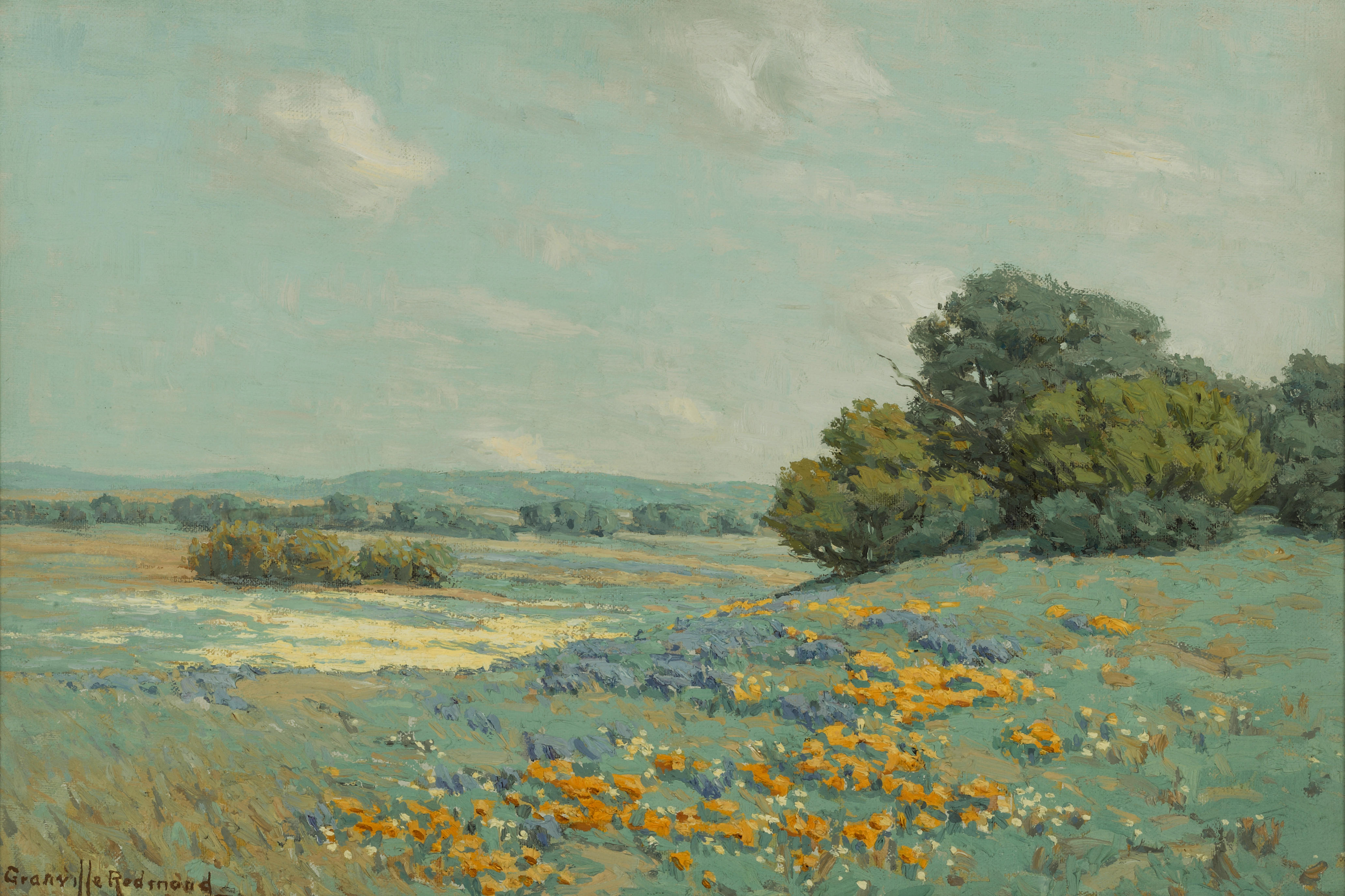This detailed painting depicts a serene landscape featuring an open, uneven field without any man-made structures. The field is primarily covered in blue-tinted grass intermixed with vibrant orange flowers. Variations in the terrain include rolling hills and valleys, dotted with light and dark green plants and taller bushes, especially on the right side. Some portions of the field appear cream-colored, adding to the diversity of the landscape. In the farther distance, clusters of trees with varying shades of green create a sense of depth. The sky overhead is a turquoise blue with grey clouds, presenting a hazy atmosphere. At the very bottom left corner, the artist's name, "Granville Redmond," is signed in dark brown, affirming the artwork's authenticity. The painting, likely done in oil, captures the tranquil essence of nature beautifully.